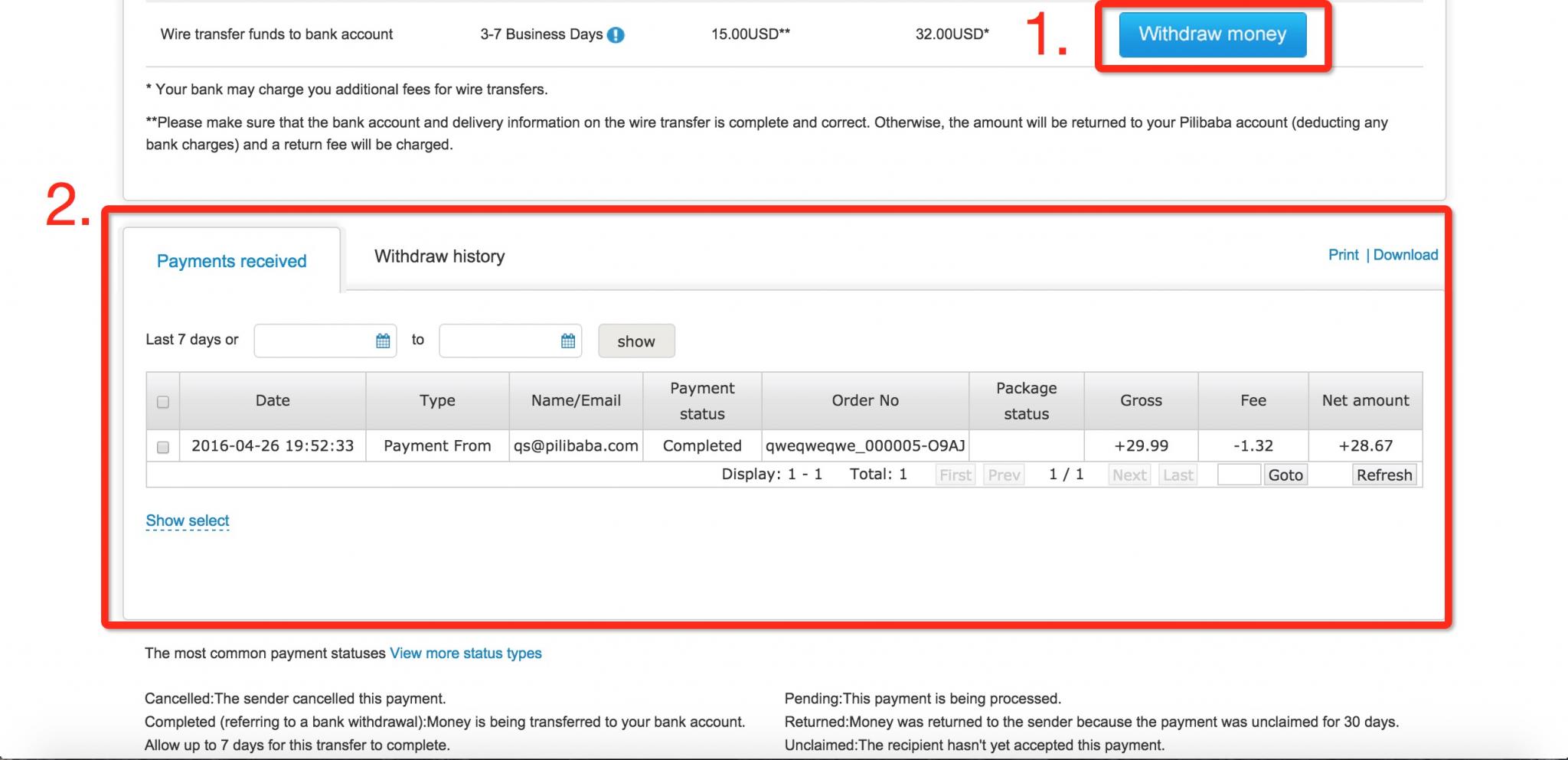A person is in the process of setting up a fund withdrawal. At the top of the interface, multiple options are visible including the option to wire transfer funds to a bank account, which takes 3-7 business days. There's a blue "More Information" button to the right of this description, which probably contains additional details, including fees of $15 and $32 marked with asterisks. To the right of this section, there's a prominent red number "1" and a blue "Withdraw Money" button outlined in red. 

Beneath this, a disclaimer notes that the user's bank may charge additional fees for the wire transfer, and advises ensuring all wire transfer details are complete and correct.

Moving on to Step 2, the interface displays two tabs: "Payment Received" and "Withdrawal History". Currently, "Payment Received" is active. There are print and download options on the right. Under the "Payment Received" tab, there are two fields to fill out: one for the last number of days, which includes a calendar function, and a "Show" button to the right of these fields.

Below this are columns labeled Date, Type, Name and Email, Payment Status, Order Number, Package Status, Gross, Fee, and Net Amount. Currently displayed is a payment dated 04-26 at 19:52. The type is "Payment Form", with the email and a payment status of "Complete." The order number is filled in but the package status is blank. The gross amount is $29.99, with a fee of $1.32, resulting in a net amount of $28.67. The display shows 101 items and has a "Show Select" button in blue.

Below all these details, there's a note outside the box explaining the most common payment statuses, including pending and unclaimed, among other types.